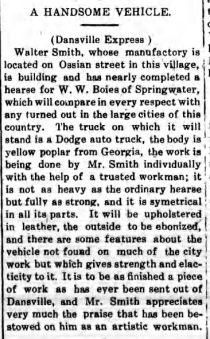This image is a scanned photo of a newspaper clipping titled "A Handsome Vehicle" by Dansville Express, with a white background and black text framed by vertical black lines on each side. The article details the nearly completed hearse being built by Walter Smith, whose manufacturing is located on Osceola Street in the village. The vehicle is being constructed for WW Boys of Springwater and promises to match the quality of any from large cities in the country. The hearse's body is made of yellow poplar from Georgia and is mounted on a Dodge auto truck. The construction is overseen personally by Mr. Smith with the assistance of a trusted workman. Notably, the hearse is lighter yet just as strong as conventional hearses, boasting symmetry in all its components. It will be upholstered in leather, with the exterior being either embonized or galvanized, and includes unique features that enhance its strength and elasticity, setting it apart from typical city productions. This hearse is described as one of the finest pieces to ever come out of Dansville, reflecting the high praise and artistic recognition Mr. Smith has received for his craftsmanship.